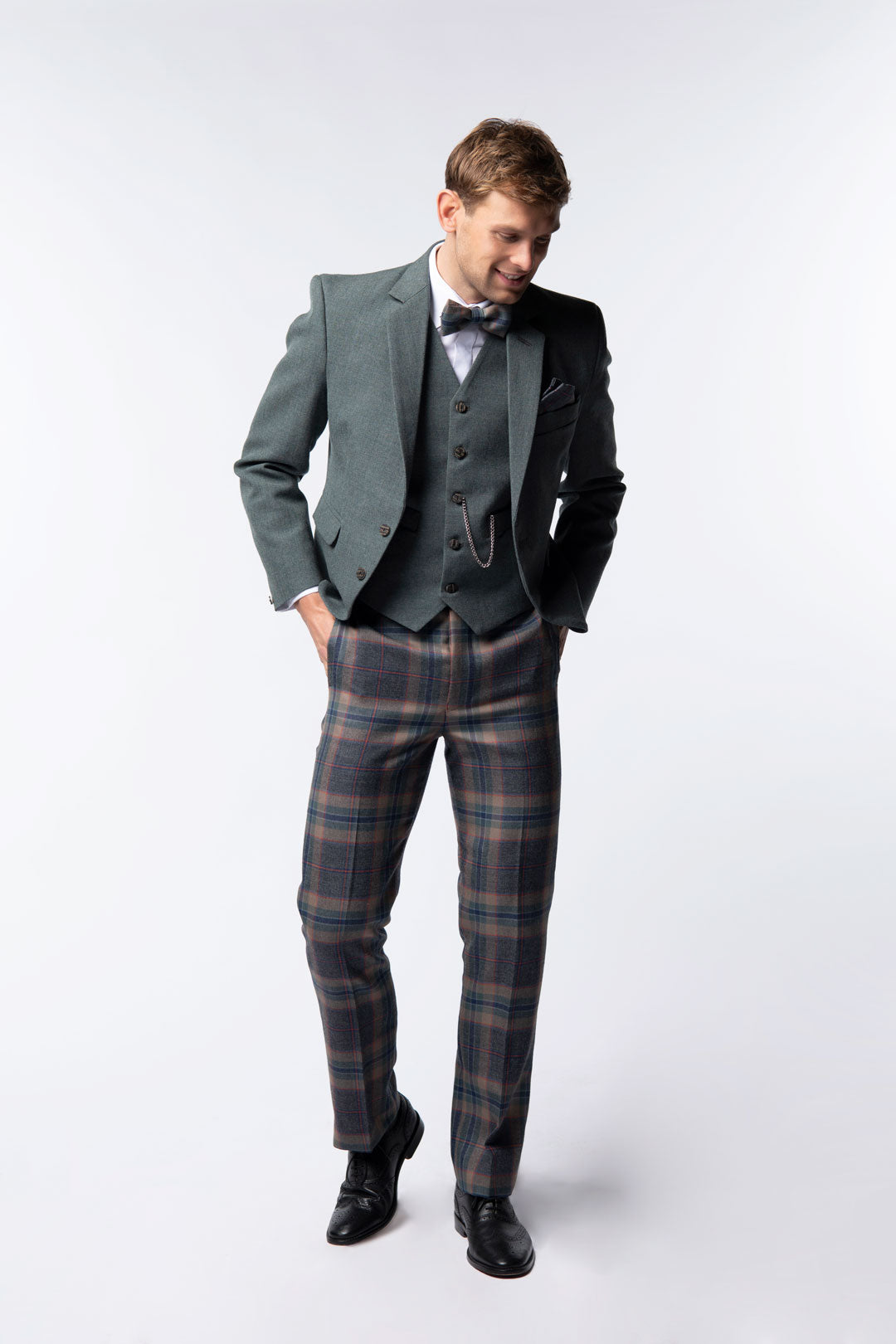This image features a young, fair-skinned man with short, neatly combed brown hair, standing against a white or potentially transparent gray background. He is dressed in a modern but vintage-inspired outfit. The focal point of his attire is a coordinated gray three-piece suit consisting of a well-fitted gray vest with buttons down the front, a matching suit jacket with two front buttons and pocket flaps, and a neatly folded light or gray handkerchief in the breast pocket. Complementing his vest and jacket is a white button-up shirt and a matching gray bow tie. He adds a touch of classic elegance with a pocket watch chain, intricately draped from the vest.

His lower half features striking plaid pants in shades of gray, blue, red, and tan. The plaid pattern also includes dark greens and dark purples with red pinstripes, creating a visually engaging contrast with his more muted upper attire. His shiny black leather dress shoes further elevate his sophisticated appearance.

The man is captured mid-step, with his hands casually placed in the pockets of his tailored pants. His posture is relaxed as he looks downward with a faint, soft smile on his clean-shaven face, possibly indicating a subtle afternoon shadow. He exudes a gentle confidence and a timeless charm, striking a perfect balance between contemporary fashion and vintage elegance. There is no text in the image.